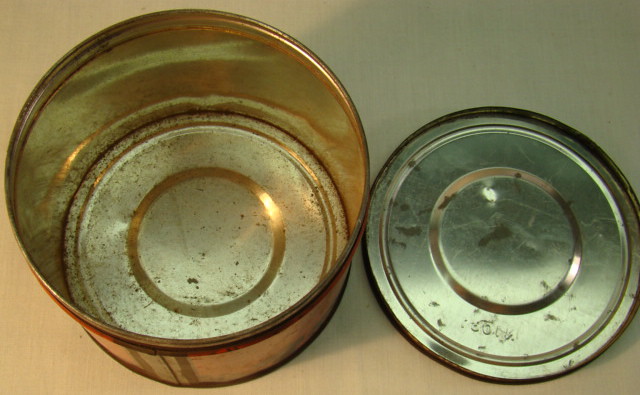This digital photograph, likely taken indoors, features a relatively large, silver-colored tin can and its accompanying lid against a textured background that appears off-white, grayish, or slightly yellowish in hue, possibly resembling a tablecloth. Both the can and its lid are shown open, positioned centrally with the lid to the right of the can. The interior of the can is notably dirty, with visible leftover dirt or black spots scattered at the bottom, suggesting it had contained something previously or had been left open for a while. The lid, which also displays a small circle on its inner surface, bears an indent and possibly some numbers, potentially indicating a manufacturing or lot number. A white reflection, likely from a light source or a camera flash, is noticeable in the upper part of the image, adding to the detailed representation of this metallic object scene.